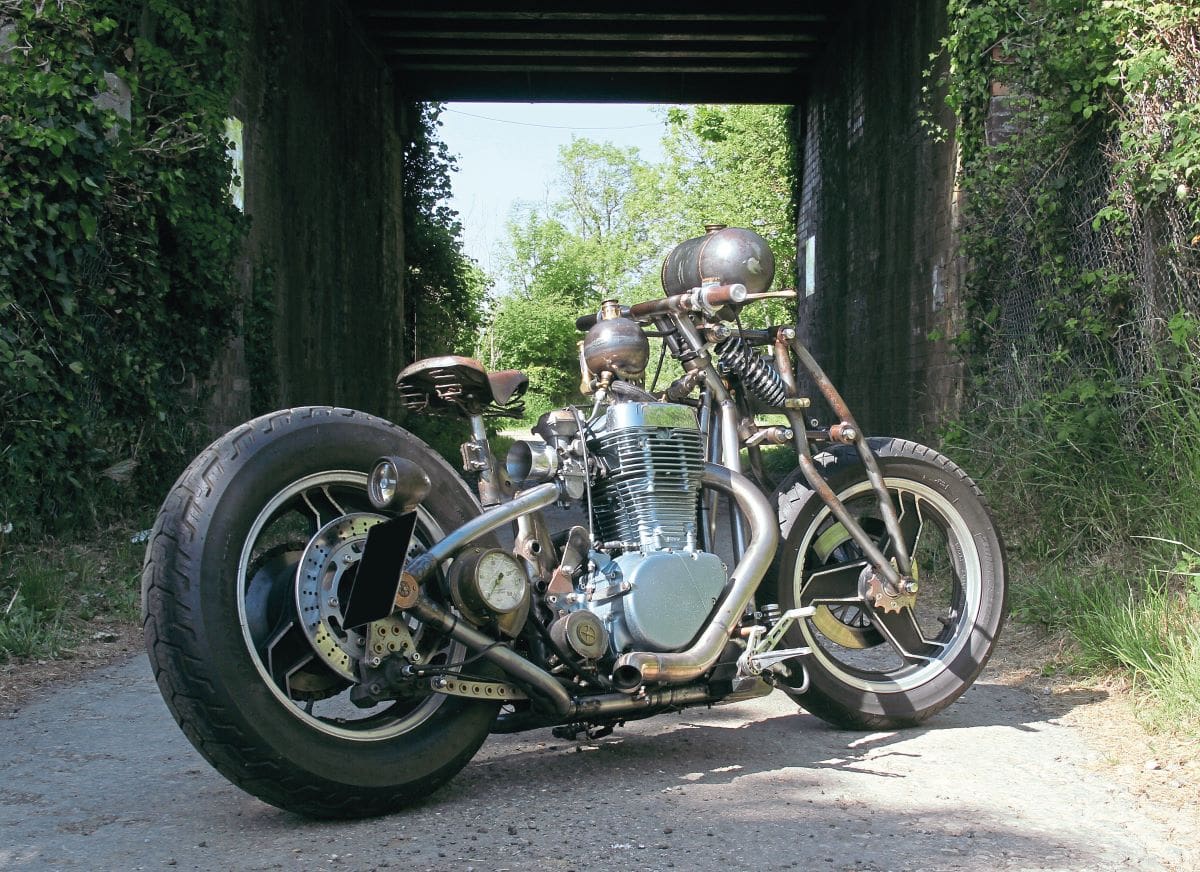This outdoor photograph captures a striking scene centered around a unique steampunk-inspired motorcycle parked on a light gray cement pathway. The motorcycle boasts a striking design with a mix of chrome engine parts and bronze-tinged handlebars. Accentuating its eclectic charm, there is a quirky water boiling steamer and an array of slightly rusted silver pipes. The bike's seating is a rich brown leather, while its tires, an oversized black rear tire, and a smaller front tire, hint at its imposing presence. The setting is lush with greenery: ivy-like leaves cover both a stone wall on the left and a chain-link fence on the right. Adding depth to the image, there's a bridge in the background, framed by trees and a clear sky, all drenched in sunlight. The scene effortlessly blends nature with an industrial aesthetic, making the photograph visually compelling.